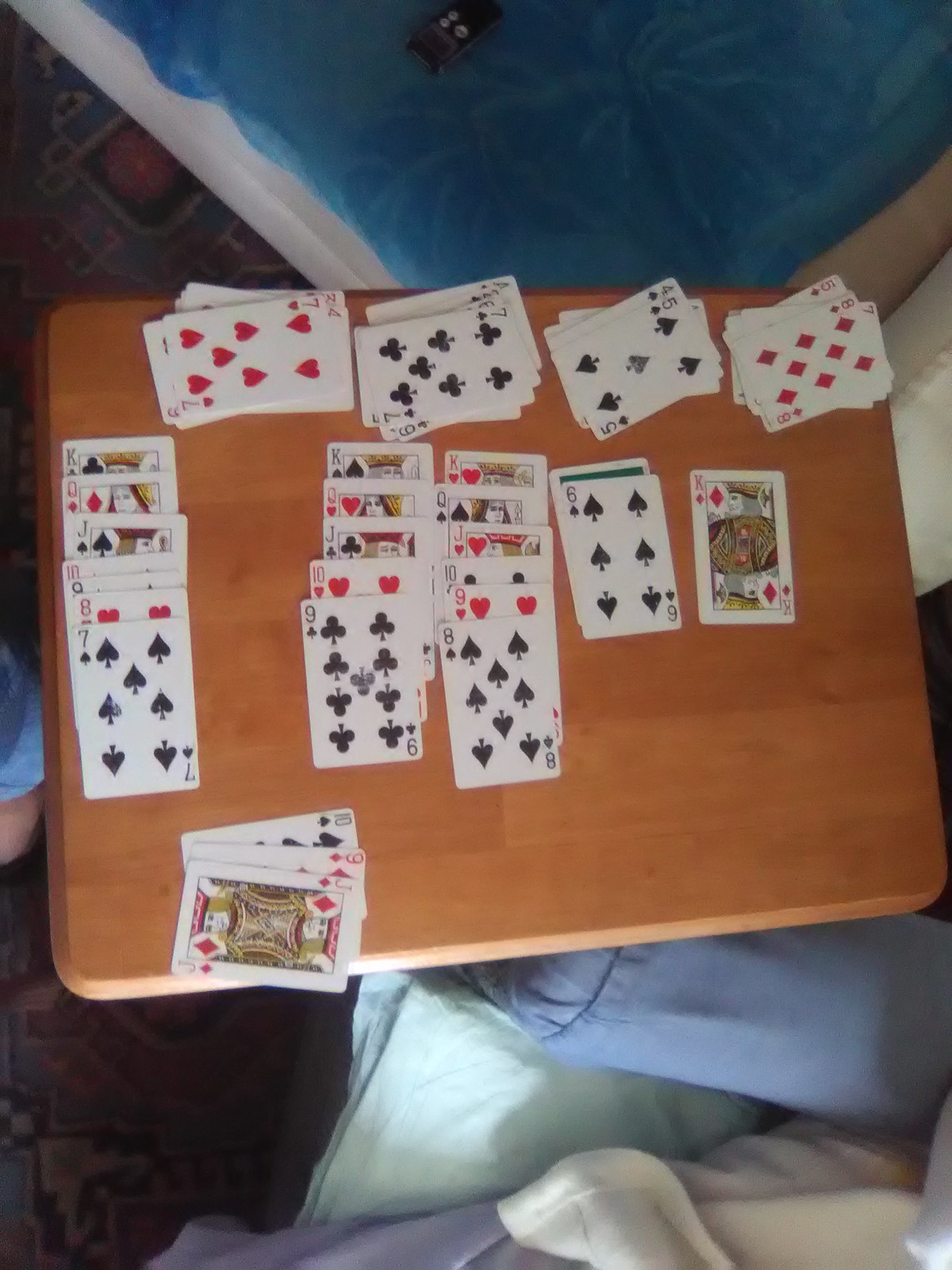The image depicts a serene, bird's-eye view of a small, rectangular brown table set up for a game of solitaire. The table is located in the center of the image, surrounded by cozy, soft furnishings. At the bottom of the image, there are neatly arranged bed linens or blankets in shades of blue, white, and green, creating a tranquil and inviting atmosphere. The top of the image offers a glimpse of what appears to be a clear space, possibly part of the bedroom.

On the table, the game of solitaire is in full swing, with five rows of cards meticulously laid out. At the very top of the table, four horizontal piles of cards are positioned in the middle, extending towards the right. These piles are neatly aligned and vary in size, each featuring anywhere from one to six cards. In the bottom left corner of the table, there is a final, smaller pile, consisting of only three or four cards.

The floor surrounding the table is adorned with a carpet featuring a repetitive emblem design in red and blue hues. Though the design details are somewhat obscured, it adds a touch of elegance to the setting. Additionally, there appears to be a remote control casually placed at the foot of the bed, hinting at the room's daily use and comfort. The overall ambiance is peaceful, with the bed's blue cover suggesting a sense of calm, reminiscent of a waterbed style.